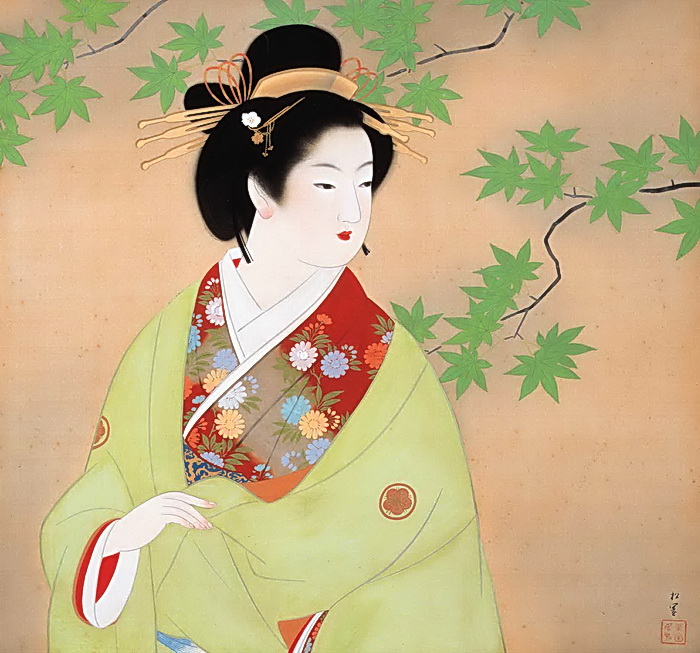The image depicts a beautifully detailed, artistic rendition of a traditional Japanese geisha woman centered slightly to the left, oriented looking down and to the left. Her skin is white, adorned with small red lips and black hair elegantly styled up with light brown clips decorated with white and brown flowers. The woman is wearing a light green robe over a traditional Japanese dress, which features a vibrant array of blue, yellow, pink, and orange flowers on a red background with a white undershirt. Her overall appearance is both serene and intense. The background comprises a tan beige wall, delicately adorned with scattered green leaves and black branches. The artwork, possibly a painting or a color pencil drawing, vividly captures the beauty and traditional elements of the geisha, combining smooth, pretty facial features with intricately detailed clothing and surroundings.